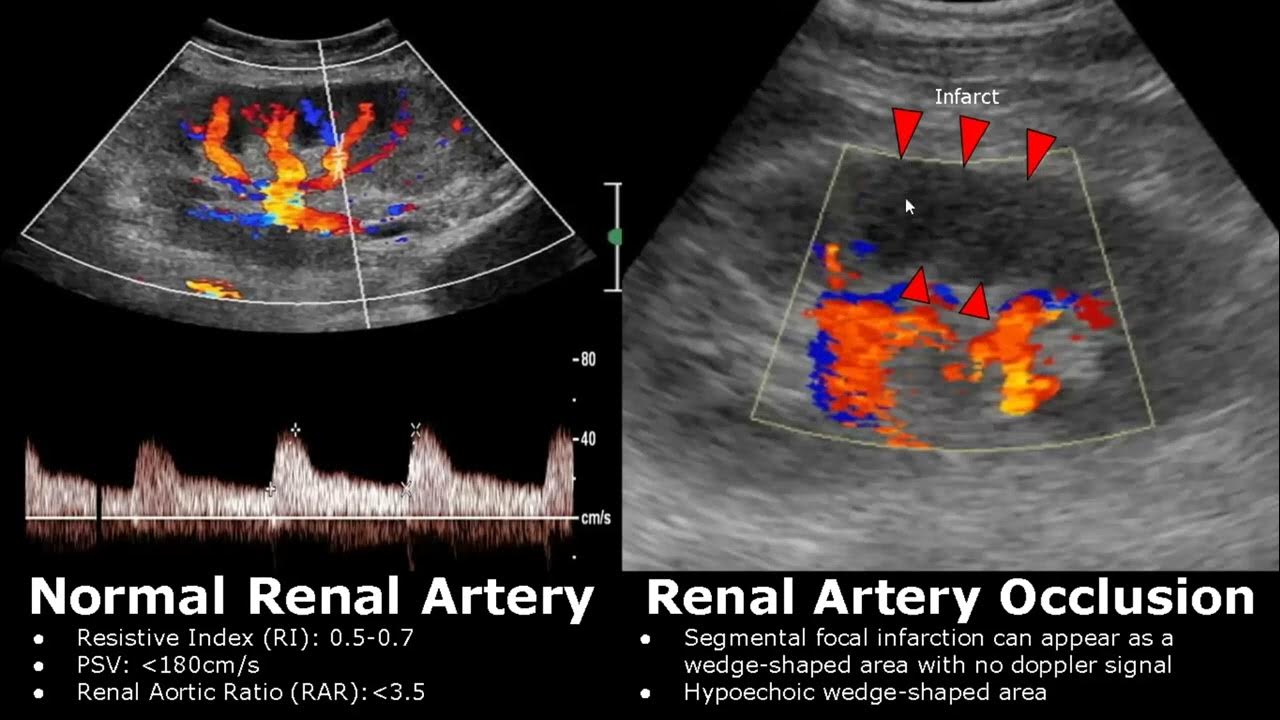This detailed descriptive caption is for a color-coded ultrasound infographic, comparing normal renal artery and renal artery occlusion. 

On the left, the image is labeled as "Normal Renal Artery." Key metrics are displayed: a resistive index (RI) ranging from 0.5 to 0.7, a peak systolic velocity (PSV) of less than 180 cm/s, and a renal aortic ratio (RAR) under 3.5. The colors—red, yellow, orange, and blue—highlight different levels of activity within the artery.

On the right, the image is labeled "Renal Artery Occlusion," indicating a condition where a segmental focal infarction is present. This appears as a hypoechoic wedge-shaped area with no Doppler signal, denoting an area of infarct. The color scheme similarly uses reds, yellows, oranges, and blues to identify areas with differing Doppler signal activities.